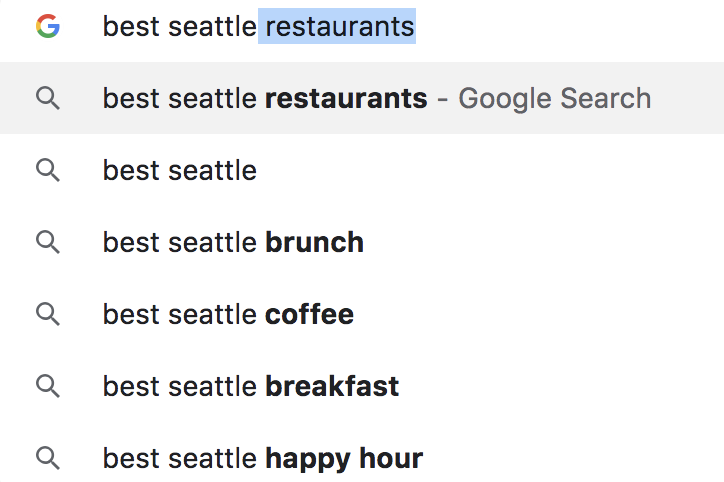The image features a white background prominently displaying the Google logo at the top. Below this, the text "Best Seattle Restaurants" is shown, with the word "Restaurants" highlighted in blue and appearing in bold font. This text serves as an example of a Google search query. The entire section containing this query is shaded in a light blue or light gray color, giving it a distinct, highlighted appearance. 

To the left of each search query is a magnifying glass icon, indicating the search function. Below the main query, there is a list of related search suggestions:

1. "Best Seattle" 
2. "Best Seattle Brunch" (where "Brunch" is bold)
3. "Best Seattle Coffee" (where "Coffee" is bold)
4. "Best Seattle Breakfast" (where "Breakfast" is bold)
5. "Best Seattle Happy Hour" (where "Happy Hour" is bold)

These suggestions are displayed as potential follow-up searches, with each keyword emphasizing the specificity of the search topic in bold font for better visual hierarchy.